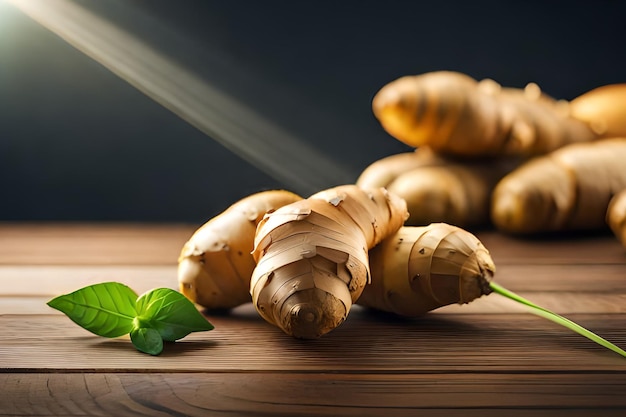This high-quality digital art image features a wooden brown-colored table at the bottom, showcasing a detailed arrangement of ginger roots. At the center sits a prominent brown ginger, with three vibrant green leaves positioned to its left. From the end of this central ginger, a long, slender green stem emerges. Behind it, to the right, there is another ginger that appears blurred, indicating depth and focus effects. Additionally, a pile of these gingers is visible in the background, also slightly blurry, further enhancing the image's depth. The background is a stark black, highlighting the main subjects, with rays of light seemingly emanating from the top left corner, casting a gentle glow onto the gingers and enhancing their flaky, textured surfaces. The composition suggests these roots are ready for culinary use, displayed artfully on the light brown wooden platform.